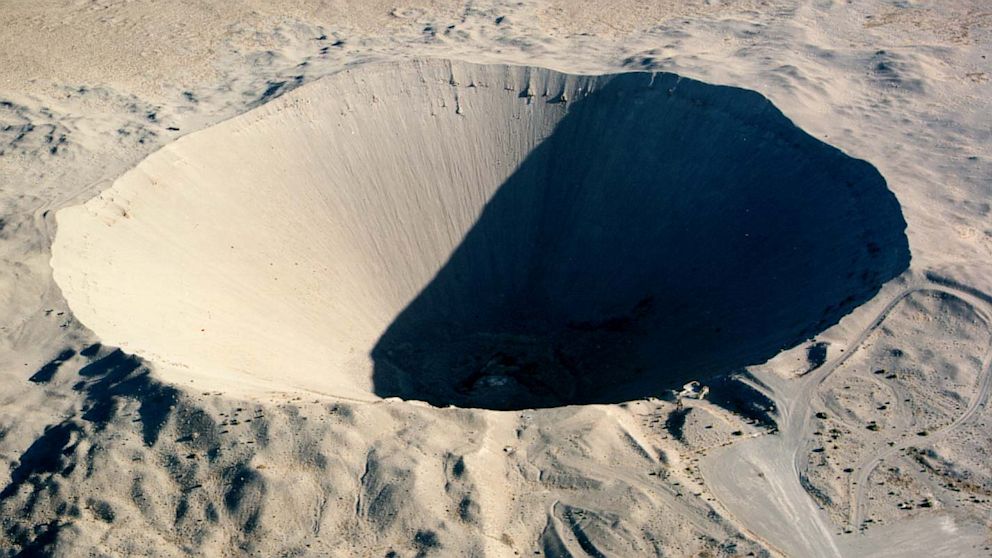This aerial photograph captures a vast, almost perfectly circular impact crater set in an expansive desert landscape, which spans approximately 1.5 times wider than it is tall. The image, likely taken from a drone or helicopter, showcases a predominantly sandy terrain with noticeable roadways visible on the right-hand side, hinting at a significant altitude. The crater itself is estimated to be 200-300 feet deep, marked by concentric striations in the sand that slope inward, forming a conical depression. The lighting is sourced from the right, illuminating the left side of the crater while casting substantial shadows on the right, obscuring complete visibility. The central area of the crater contains indistinct structures that might be a building or a research facility, particularly notable in the parts cloaked in shadow. Additionally, there is a peculiar greenish glow at the base that could suggest the presence of water or some other natural substance. This large-scale image distinctly highlights the desert's characteristic dunes and hills, integral to the crater's dramatic and isolated setting.